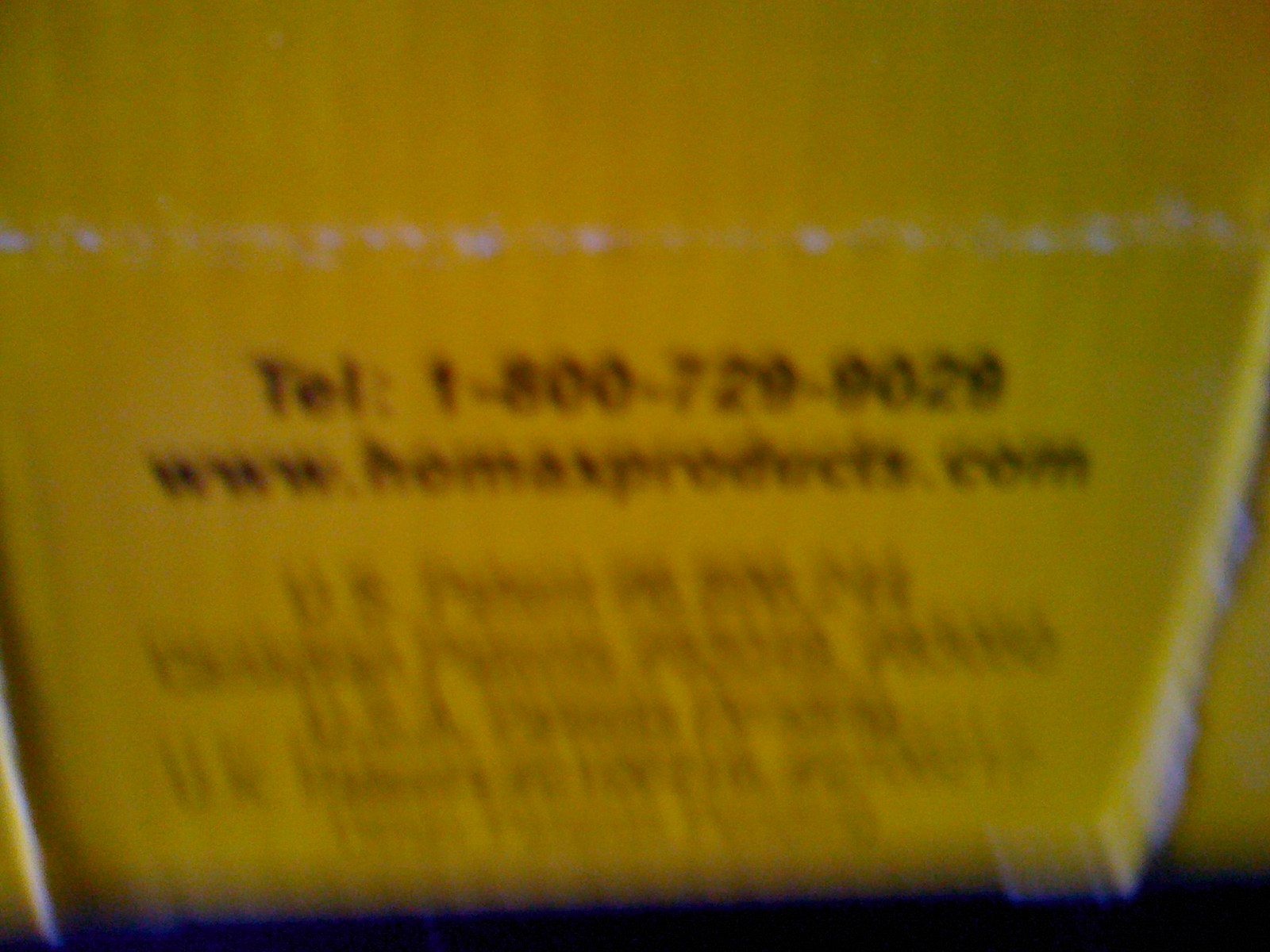This image presents a wide but horizontally narrow composition, featuring an out-of-focus view of a yellow object adorned with text. The image is taken from an elevated angle, causing the object to appear foreshortened; it is wider at the top and tapers towards the bottom. The primary visual elements include a strip of black at the base of the object with a bluish-purple line at the very bottom, giving a sense of depth and shadow. 

In the middle of the yellow object, there is black text that is partially legible. The words 'tell,' akin to 'telephone call,' are somewhat decipherable, followed by a phone number, 1-800-729-9029. Below the phone number, in smaller text, a website is listed, which appears to be www.homexproducts.com, though the exact URL is indistinct. At the very bottom of the object, additional text begins with 'US,' but the details are too blurred to be readable.

The top of the object features a white line, possibly indicative of a border or a reflection of light. The background remains largely dark and shadowy, adding contrast to the brightly colored and text-laden main subject.